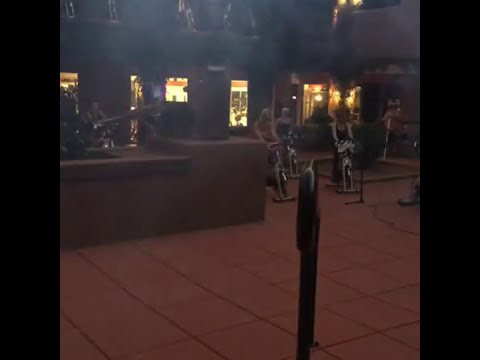The photograph, taken at night, exhibits a smoky, dark ambiance, and seems to capture an outdoor patio area. Red clay tiles cover the ground, giving it a classic patio feel. Central to the scene are three women exercising on stationary bikes, slightly blurred and enveloped in a misty atmosphere. To the left, a multi-layered garden structure with a brick retaining wall is seen, housing some plants. In the background, illuminated by a warm yellow glow, stand glass doors and windows, possibly leading to a gym or store, hinting at a commercial context. Columns supporting an overhang add to the architectural complexity, making the scene resemble a movie set. Despite the blurriness and the dark conditions, the overall mood is vibrant and dynamic, with hints of exercise and leisure intertwined.